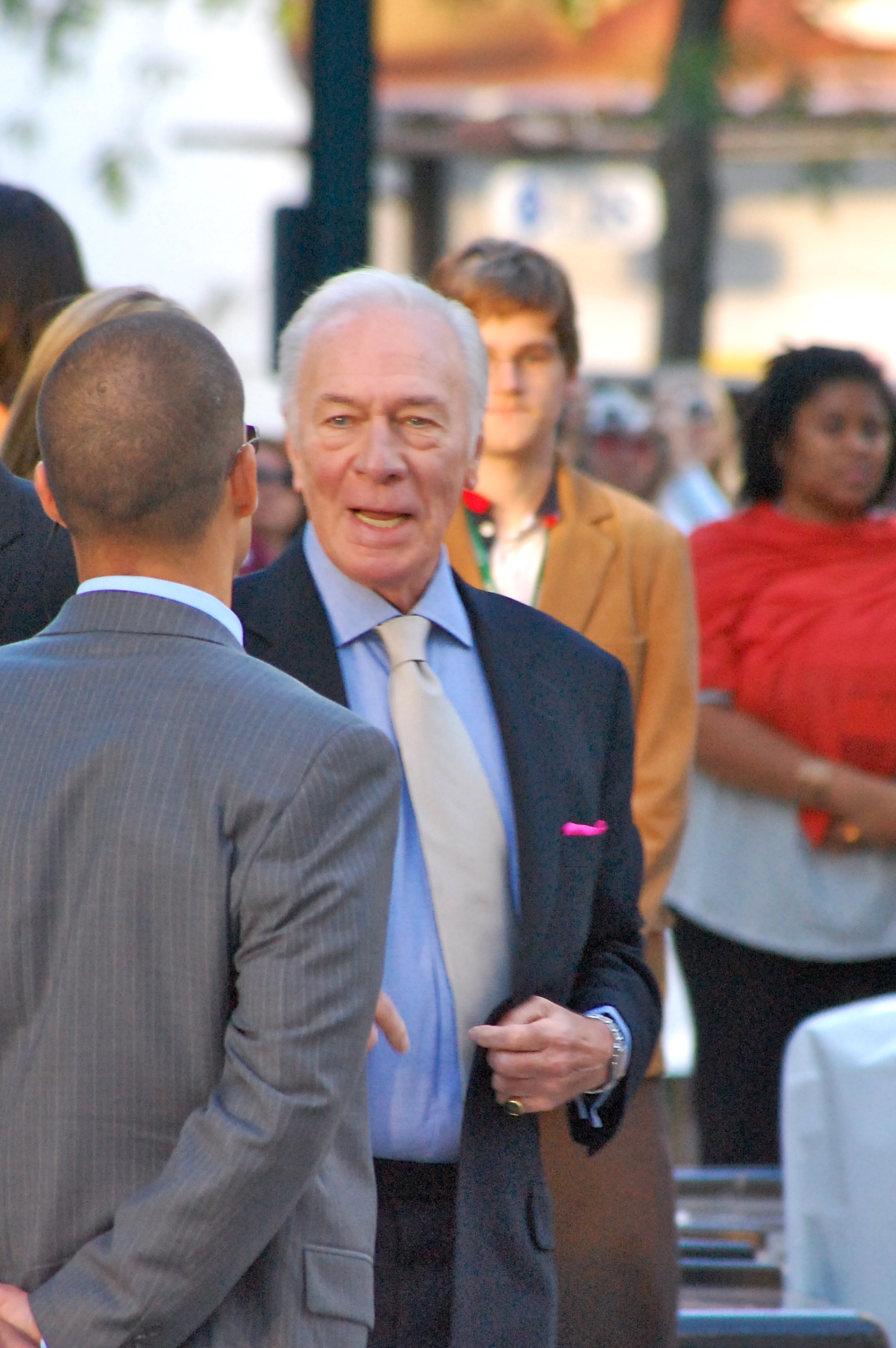In the center of the image, an older gentleman identified as Christopher Plummer is seen talking to another man who is slightly off to the left. Christopher Plummer is dressed in a dark blue suit jacket, a light blue shirt, and a light beige tie. He also sports a bright pink pocket square. The man he is conversing with has his back to the camera; he is wearing a gray pinstripe suit and has a short buzz cut hairstyle. 

In the slightly out-of-focus background, there is a crowd of people who appear to be staring at Christopher Plummer. Among them, directly behind Plummer, stands a man with short brown hair, glasses, and a tan (naugahyde color) suit jacket. To the right of this man is a black woman dressed in black pants, a gray shirt, and an orange shawl draped over her chest. The far background remains blurry, featuring indistinct elements that might be tree trunks or building posts.